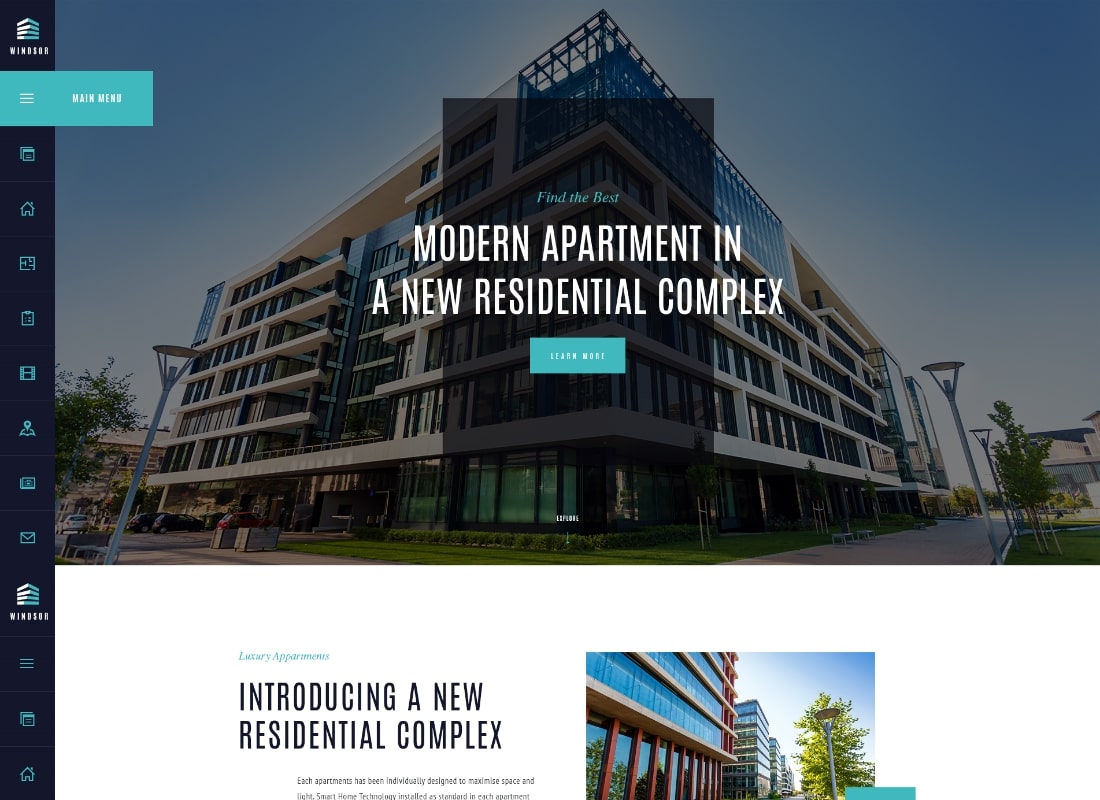This vertical and horizontal image appears to be a screenshot of a web page likely viewed on a computer monitor. The page features a simplistic design, utilizing the white background of the screen itself. 

On the left-hand side, there is a navy-blue vertical sidebar adorned with various clickable icons. The standout icon is the second one from the top, which consists of three horizontal lines and a "Main Menu" label against a sage-green background.

The central section of the webpage showcases a photograph of an apartment complex. The picture features a clear blue sky, a large modern building, several trees, and streetlights. Overlay text in white reads "Modern apartment in a new residential complex," with an option to click for more information.

At the bottom of the page, there is an introductory section that announces the new residential complex. This section contains a brief description in black text. Below this, there is another image focusing on several floors of the apartment building, accompanied by a tree and a streetlamp, further emphasizing the modern and serene ambiance of the complex.